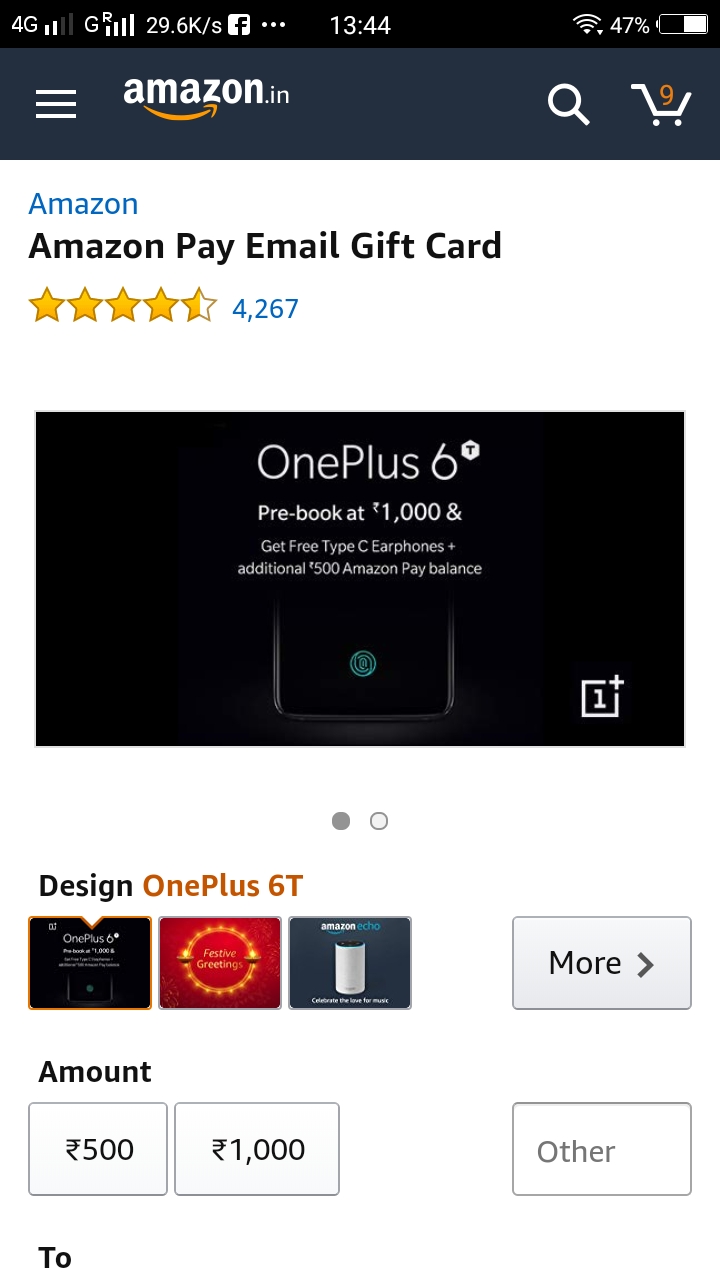The image is a vertically oriented screenshot taken on a mobile device. At the very top, a thin black bar displays standard status indicators such as "4G," the data transfer speed "29.6K/s," the Facebook icon, the time "13:44," and a battery level of 47%. 

Below this, there is a dark gray horizontal bar indicating that the user is on the Amazon.in site, with a cart icon showing nine items. 

Underneath this bar, you'll find the Amazon branding in blue followed by "Amazon Pay Email Gift Card." This item has garnered 4,267 reviews, boasting an impressive average rating of 4.5 out of 5 stars. 

Below this information, an image of the gift card comes into view. The gift card itself appears as a black rectangle, linked to a promotion for the OnePlus 6. The promotion details reveal that pre-booking the device for 1,000 rupees entitles the buyer to free Type-C earphones and an additional 500 rupee Amazon Pay balance.

Further down, the lower part of a black phone is visible. The phone's screen displays a green thumbprint symbol, and the caption "Design OnePlus 6T" is prominently featured. Three design options are illustrated next: a black phone, a red phone, and an option labeled "Amazon Echo" with an accompanying image of the Amazon Echo device. 

Lastly, two amount options for the gift card are shown: 500 rupees and 1,000 rupees.